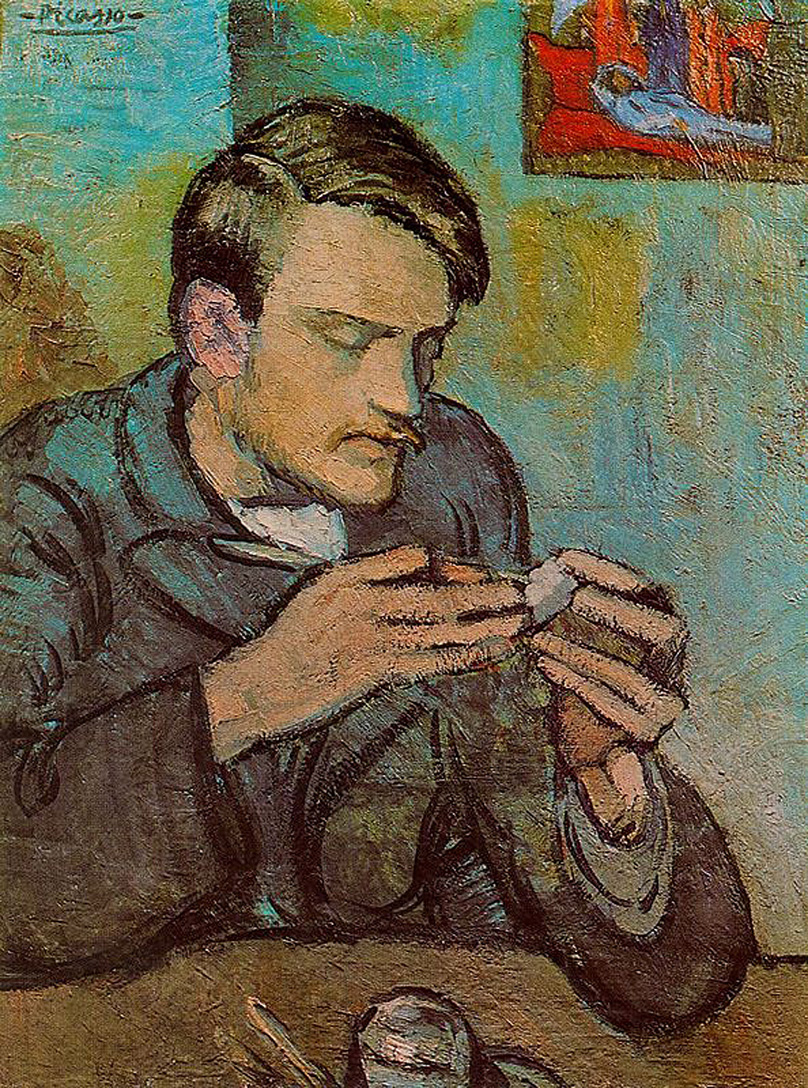The image is a detailed painting of a man seated at a brown table. The man, with neatly parted short brown hair and a light brown mustache, has his eyes half-closed as he intently stares at a grey item in his hands. He is dressed in a bluish-grey suit jacket over a white shirt. His right hand holds a crafting tool, while his left cradles the grey object, which appears to be a pipe that he is examining or filling. Behind the man, the wall features a blue, yellow, and brown splotched pattern. In the upper right corner of the painting, there is a smaller picture depicting a person lying on a red bed with drapes in the background. An inscription at the bottom left of the image reads "Picasso," indicating the artist. The colors in the painting range from black, white, grey, and brown to shades of blue, red, orange, and purple.